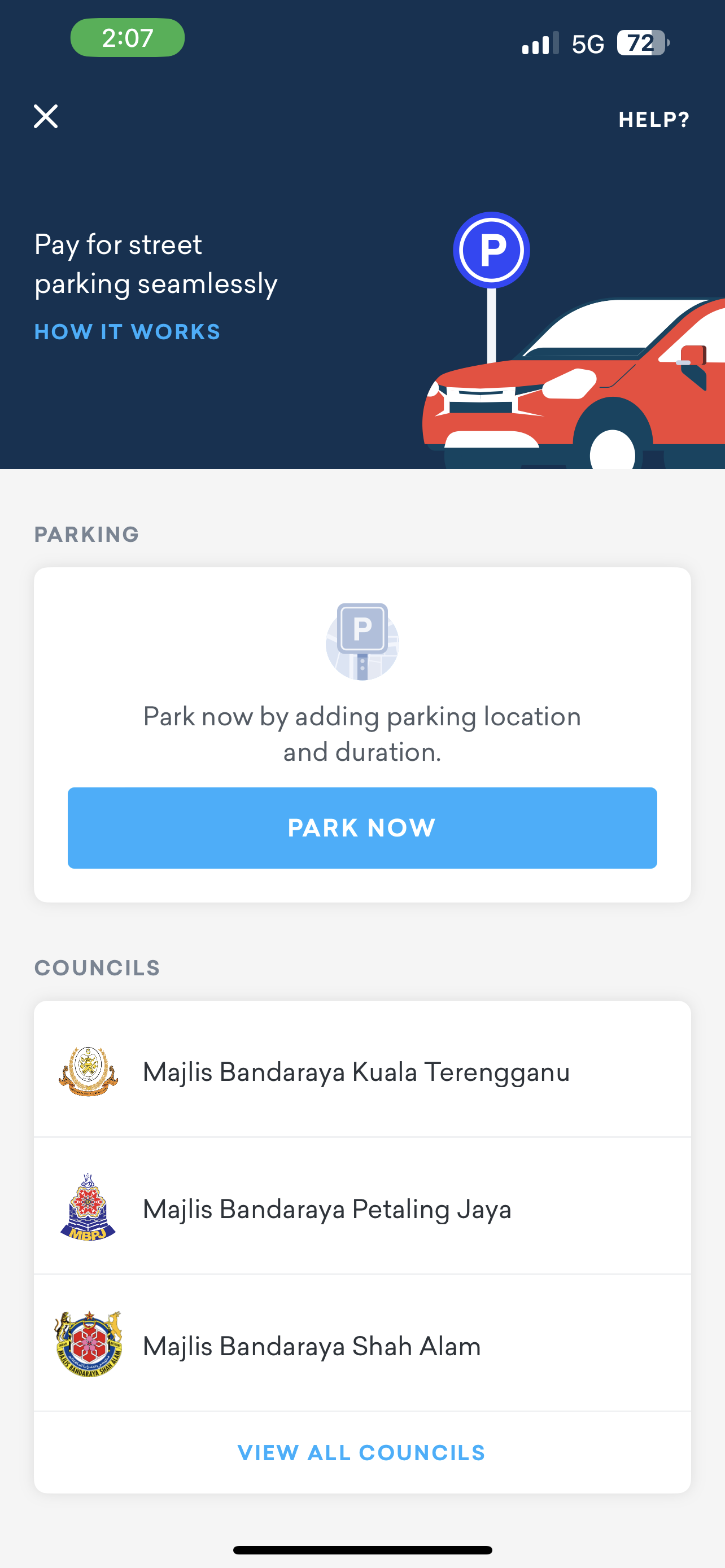This screenshot captures a smartphone interface themed with a navy blue header at the top. In the upper left corner, a green rectangle with rounded corners displays "2:07" in white, likely indicating the current time. The upper right corner features icons showing a battery level at 72%, 5G connectivity, and signal strength with three out of four bars illuminated in white.

Below the header, a text in white reads "Pay for street parking seamlessly," followed by "How it works" in blue. On the right side, there is a simple, stylized illustration of a red car with white accents for the windshield and wheel hubs. Adjacent to the car is a blue circle with a white 'P,' denoting parking.

The background transitions to a very light gray as we move below this content. Centered, a white rectangle labeled "Parking" introduces a message: "Park now by adding parking location and duration." Below this, a turquoise blue rectangle with white font invites users to "Park Now."

Further down against the light gray background, the word "Councils" appears, followed by another white rectangle listing three council names starting with "Majlis." At the end of this list, a blue text reads "View all councils," suggesting that tapping it would reveal the full list of council names.